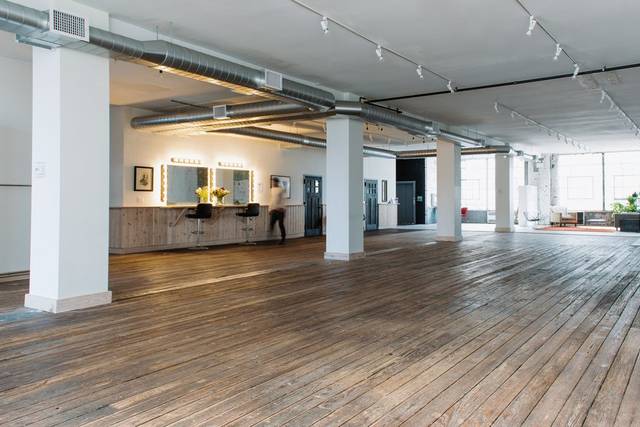This image depicts an interior of a commercial area, potentially a beauty or barber shop, featuring a cozy, low-ceilinged setup. The floor is comprised of wood slats or plank flooring, exhibiting signs of wear. Along the left wall, there are a couple of windows with two swivel chairs positioned in front, suggesting spaces where interactions, possibly makeup or hair styling sessions, occur. The room is dotted with several pillars and overhead lights, adding to the functional design of the space. In the background to the right, large windows allow natural light to flood in, while a receding area suggests additional room extending further back. A person can be seen standing towards the left, near some pictured decor on the wall, and a few doors are visible to the right, contributing to the open and inviting layout of this commercial interior.